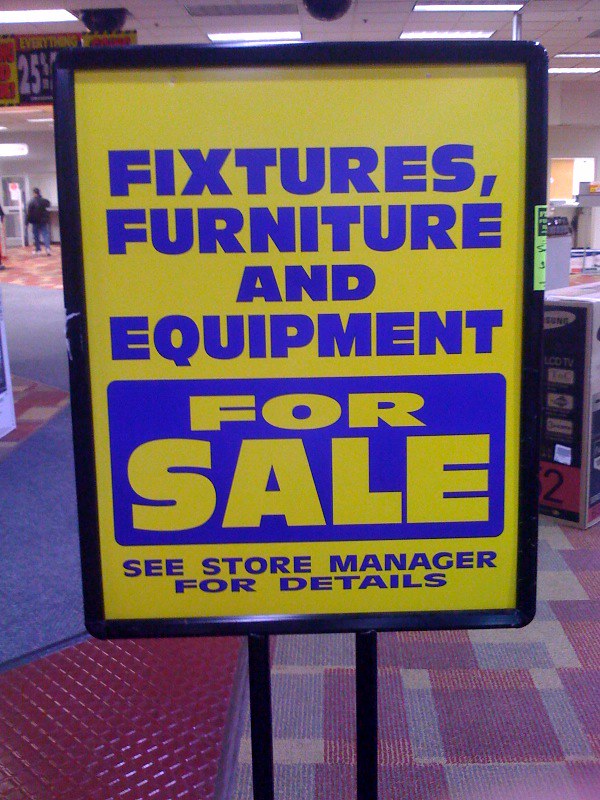The photo, taken indoors in a department store, features a prominently displayed black metal sign with a yellow background and blue lettering that reads "Fixtures, Furniture, and Equipment for Sale. See Store Manager for details." The sign dominates the center of the image. Overhead, multiple fluorescent light fixtures and fire sprinklers dot the ceiling, with a "25% off" sale sign hanging beneath them. In the background, a doorway is visible with a person walking into it. The flooring is a mix of vibrant patterns: predominantly a purple carpet with intricate gold and red geometric designs; additional sections on the right showcase checkered red and white, red plastic with ridges, blue, and grey carpets. A brown box with black sides and a red bottom sits in the right corner, along with some racks above it. To the right of the prominent sign, a box that might be for a TV stands, suggesting this could also be an electronics section within the store.